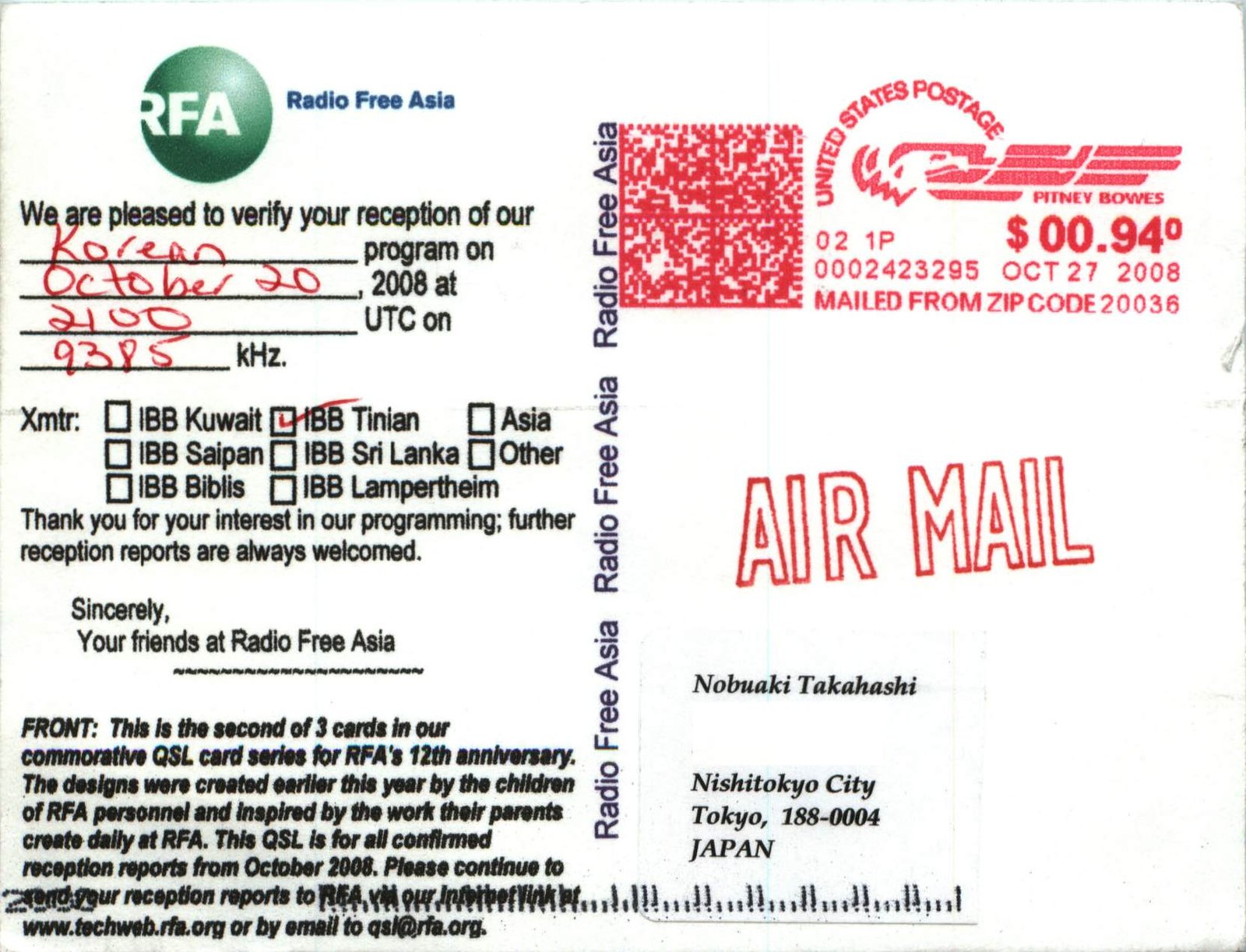The image features a landscape-oriented postcard from Radio Free Asia, prominently filling the entire frame. On the left side, in a green globe emblem with white "RFA" script, and beside it, "Radio Free Asia" is printed in blue. Below this, in black text, is a verification message for the reception of their program, thanking the recipient, Nobuaki Takahashi of Nishitoki City, Tokyo, Japan, for their interest and encouraging further reception reports. The message includes handwritten red ink details about the reception on October 20th, 2008, at 2800-2100 UTC on 9385 kHz, and a checked tick box next to "IBB Tinian." 

On the right side, a red "Air Mail" stamp and a postal indicia indicating "United States postage" of 94 cents, dated October 27, 2008, from zip code 20036, are featured. A barcode is also present. The thank-you card complements the addressed information with the structured format of a mailing postcard, showcasing colors in black, white, red, green, pink, and dark blue, resembling a photocopied print publication.